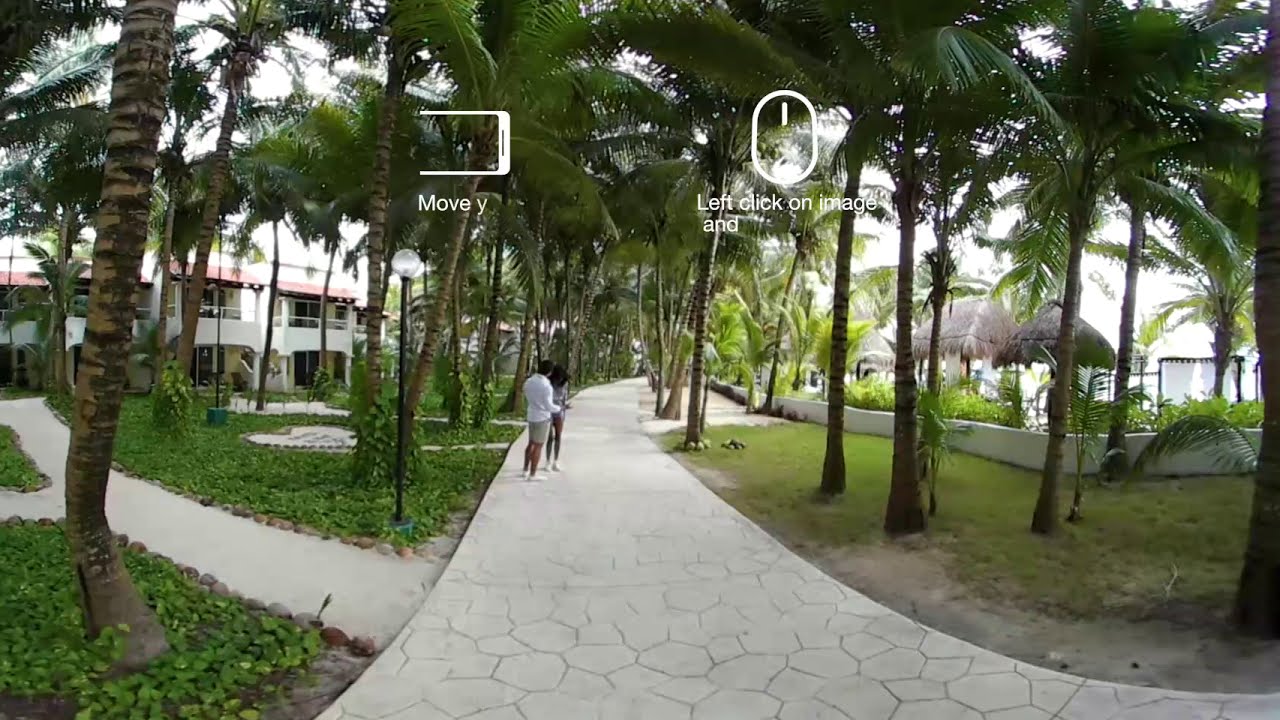This image captures a picturesque outdoor scene of a tropical resort or hotel, featuring a central stone walkway flanked by verdant palm trees and lush green plants. The path, made of cracked or tiled stones, stretches through a vibrant landscape. On the left, two-story white buildings with balconies offer views of the serene surroundings. On the right, a low stone wall supports thatched-roof huts, hinting at a relaxing retreat space. Two figures, a man in white tennis shoes, khaki shorts, and a white shirt, and a smaller individual possibly a female with dark hair, are visible halfway down the path. Overlaid on the image are interactive overlay elements: text at the top left reads "move Y" with a sideways outline of a phone, and at the top right, "left click on image" is paired with a mouse icon, suggesting the image could be part of a 360-degree panoramic view. The bright, neon-green grass and various tropical trees enhance the exotic ambiance of the scene.